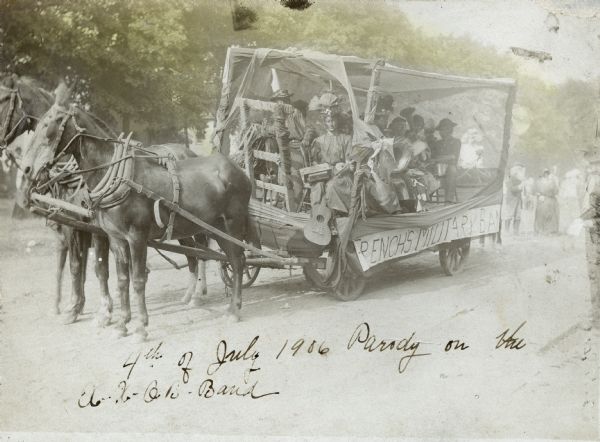This is a faded black and white (with hints of green from the background trees) historical photograph dated July 4th, 1906. It captures a stationary horse-drawn carriage, pulled by two horses adorned with ropes and blinders. The wagon is crowded with people dressed in period attire reminiscent of the 1910s or 1920s, with some wearing long robes and one individual sporting a headdress. A sign on the side of the wagon reads "French's Military Band," indicating the occupants are likely part of a musical group, as several seem to be holding instruments. Behind the wagon, there are more people dressed in similarly old-fashioned clothes, including a man with a large hat and mustache. The overall scene is dust-laden, adding to its vintage atmosphere. The bottom of the image, although quite faded, features cursive writing that reads, "4th of July, 1906, parody on the something band," suggesting a playful or satirical representation of a military band.